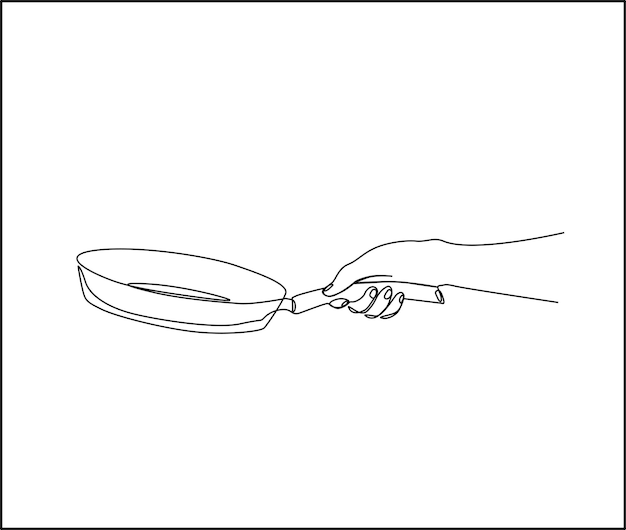This image is a simple black and white line drawing of a hand holding a frying pan, viewed from the side. The illustration features the forearm emerging from the right side, with the hand wrapping around a slightly curved handle. The hand's grip shows the top of the thumb and partial views of the other three fingers, their details outlined clearly though they lack coloring. The small frying pan, which has a thin border and a circular top, includes a short plate connecting the handle to the pan. The pan is flat with raised edges, featuring an inner oval shape. The background is entirely white, offering a clear contrast against the thin, black lines of the drawing. The entire drawing is neatly enclosed within a black border. The overall posture of the hand suggests a motion as if positioning the frying pan down.